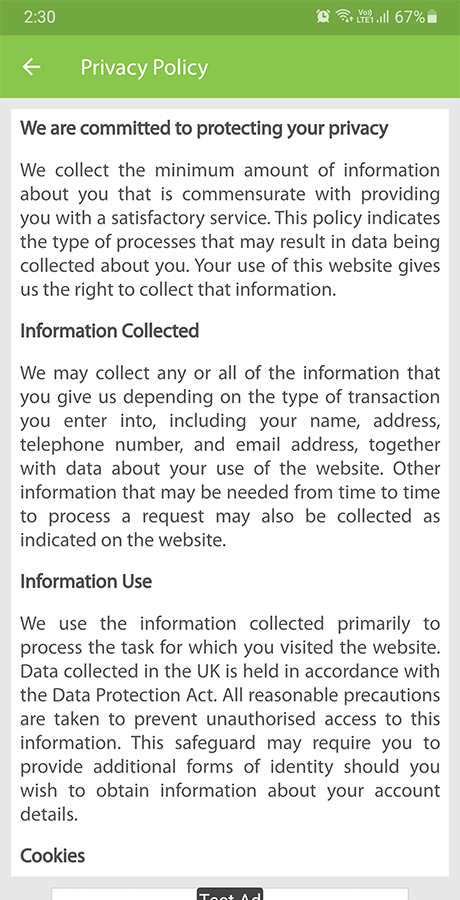This image appears to be a screenshot taken from a smartphone. The screenshot is in a vertical rectangular format. At the very top, there is a green status bar displaying the current time as 2:30 in white text on the upper left corner, along with symbols for Wi-Fi connectivity, battery level, and other typical indicators on the upper right. Beneath this, a lighter green bar contains white text reading "Privacy Policy," accompanied by a leftward-pointing arrow.

Below this header, the main content is set against a white background with black text. 

1. **Introduction Paragraph**:
   - In bold: "We are committed to protecting your privacy."
   - This section explains that only the minimum necessary personal information is collected to provide satisfactory services.

2. **Second Paragraph**:
   - In bold: "Information Collected."
   - It describes the various types of information that may be gathered based on user transactions, including name, address, telephone number, email address, and usage data of the website.

3. **Third Paragraph**:
   - In bold: "Information Use."
   - This section outlines the primary usage of the collected data, primarily for processing specific tasks related to website interaction. It also mentions that data gathered in the UK adheres to the Data Protection Act.

At the bottom left corner, the bold text "Cookies" introduces another section, but the text appears to be cut off.

Additionally, at the bottom center of the image, there is a partially visible black text which is unclear and cut off, making it difficult to ascertain its content.

Overall, this screenshot represents a privacy policy page of a website, detailing the commitments to user privacy, types of information collected, and its specific uses.